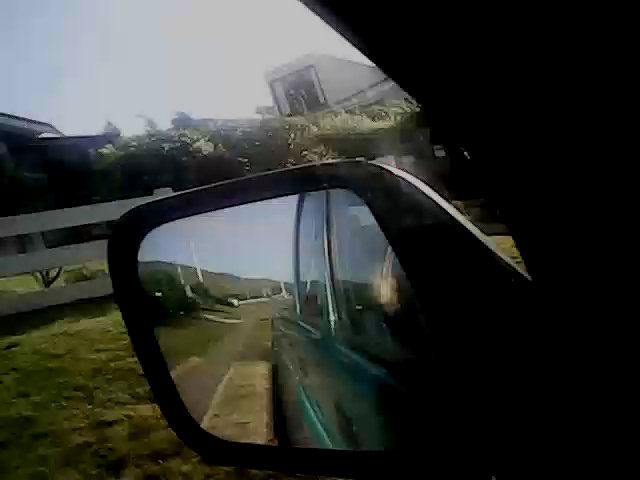The image captures the view from inside a pickup truck, focusing on the left rearview mirror. The mirror reflects a blue car behind and part of the truck's blue door, along with the window's metal separator. Beyond the mirror, the scene stretches into a vivid panorama featuring a sky that transitions from a lighter to a darker powder blue into white. The backdrop includes a white building and a white fence enclosing a yard with trees and green grass, suggesting a farm-like setting. In the distance, hills rise under the merging blue and white sky. There's also a road visible, indicating the truck is driving through this serene landscape.